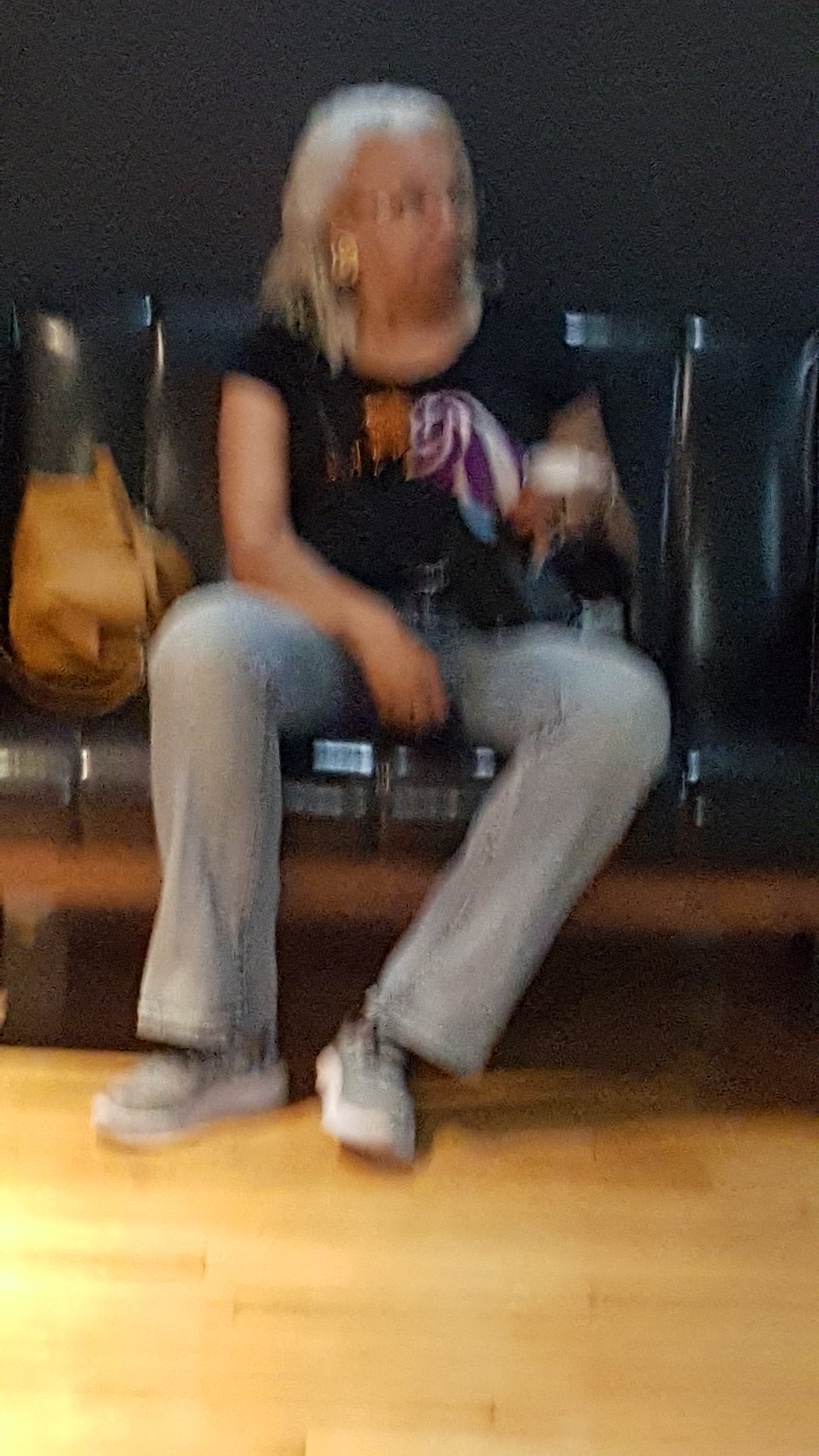A blurred photograph captures a woman seated, seemingly in motion as the picture was taken. She appears to be sitting on either a bench or perhaps stacked boxes of electronic devices. The setting includes a light wooden floor visible at the bottom, against a dark-colored wall. She is outfitted in gray, slightly loose-fitted pants paired with gray and white sneakers, and a black t-shirt adorned with a graphic design. Her white shoulder-length hair complements her large earrings and wire-rimmed glasses. One hand is raised, holding an unidentified object, while her other hand rests on her thigh. To her left, a light brown purse is visible.